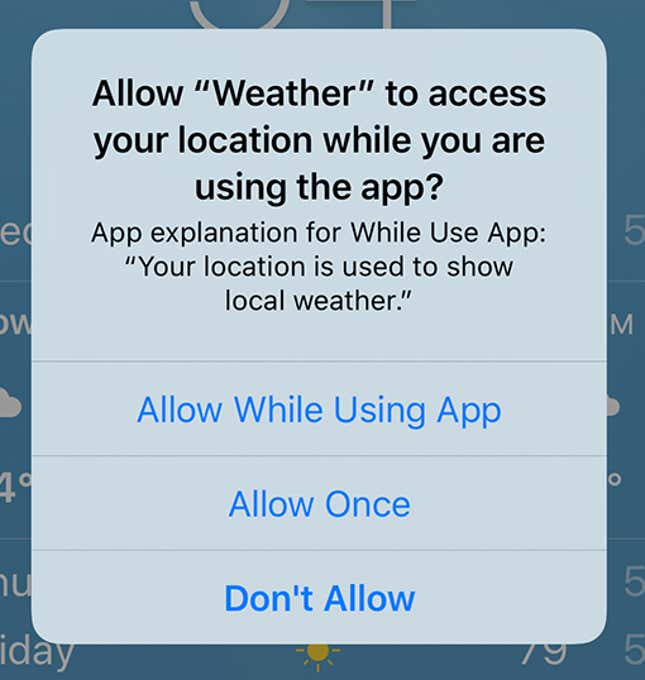The image is a screenshot from a mobile device, likely an iPhone, displaying a permission prompt from a weather app. The prompt is requesting the user's permission to access their location while using the app. It provides three options: "Allow While Using the App," "Allow Once," and "Don't Allow." All three options are highlighted in blue, with "Don't Allow" in bold, standing out more prominently. The background of the screenshot reveals a partially visible and slightly blurred weather app interface, featuring temperature readings and weather icons, though they are not clearly discernible. The prompt is designed to be straightforward and user-friendly, providing a brief explanation that the user's location is utilized to display local weather information, ensuring clarity in the choices offered to the user.